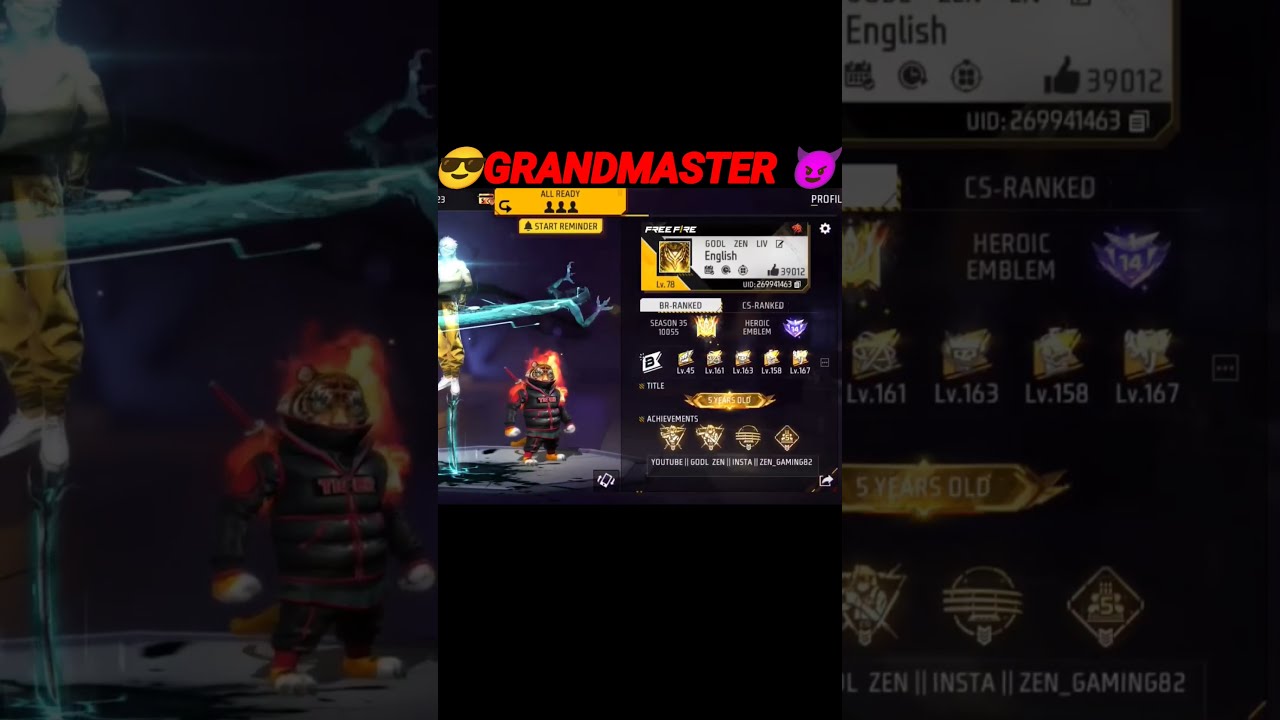The image is a detailed screenshot of a video game showcasing a high-level character profile. Centrally featured is a tiger character wearing a big puffy black coat with a red zipper, standing upright with flames behind its head and shoulders. At the top of the image, there is a smiley face emoji with sunglasses and a purple devil face emoji, flanking the red text that reads "Grandmaster." To the left of the tiger are three head icons with the text "All Ready." Below this, there's an alarm icon followed by "Start Reminder." On the right side of the image, various panels of information are displayed, including a thumbs up with the number 39012, a User ID (UID) number 269941463, and rankings such as "LS Ranked" and "Heroic Emblem." The image includes text in English, but the font size is very small, making it difficult to read additional details.